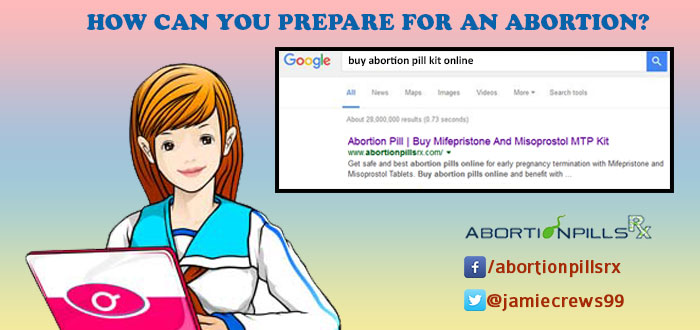The image is an advertisement for abortion pills set against a pastel-colored background transitioning from pink at the top, to blue in the middle, and beige at the bottom. On the left side, there is a detailed cartoon figure of a young woman with reddish-orange hair, wide dark eyes, and a friendly smile. She is wearing a white long-sleeved, sailor-style top with blue stripes and a red bow or scarf in the front, adding a touch of nautical charm to her appearance. In front of her is an open laptop with a pink and white cover.

At the top of the image, in blue letters, the title reads, "How Can You Prepare for an Abortion?" Below this, to the right of the woman, there is a depiction of a Google search page. The search query reads, "Buy Abortion Pill Kit Online," and the subsequent search result shown is for "abortion pill by Mifepristone and Misoprostol MTP kit," with the web address displayed below the search result.

At the bottom right of the image, there's a logo and text stating "Abortion Pills RX" along with social media handles, including a Facebook link "Abortion Pills RX" and a Twitter handle "@JamieCruz99."